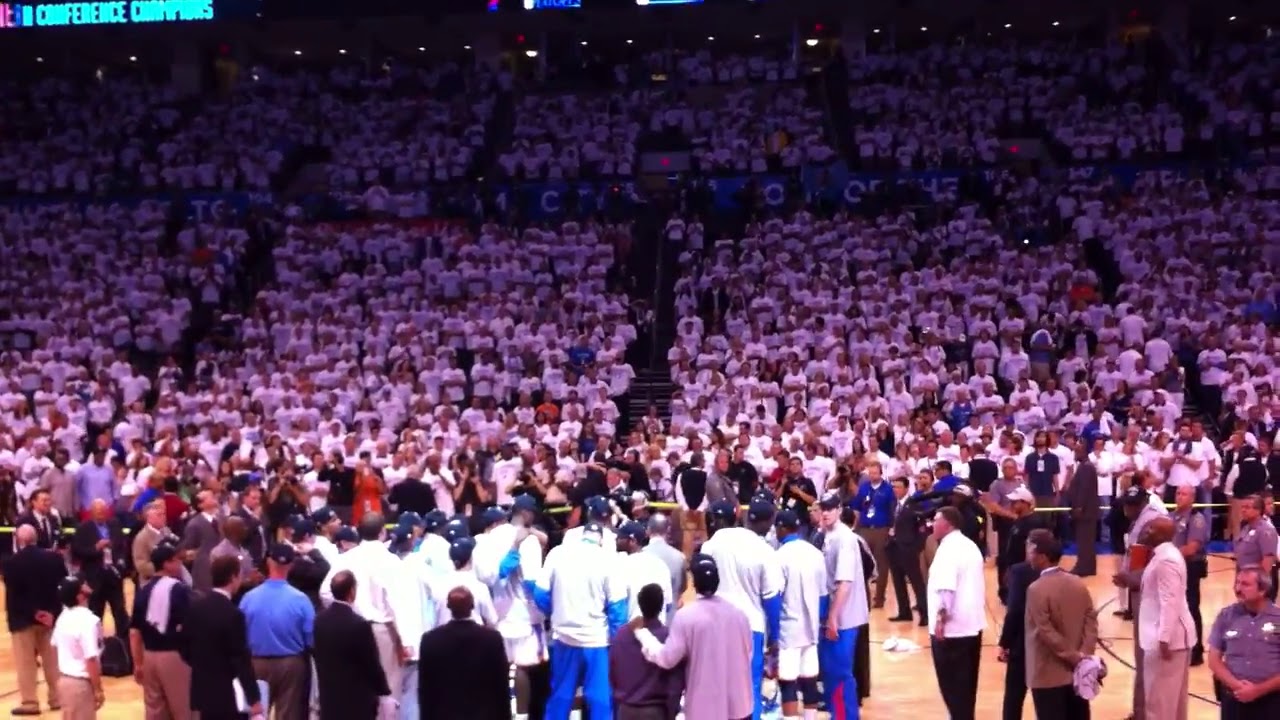The image captures a vibrant celebratory scene inside a bustling basketball arena. The horizontally aligned rectangular picture prominently showcases a densely packed crowd in the stands, which takes up almost the entire upper half of the image. The spectators, dressed predominantly in white t-shirts, create a sea of white that underscores the festive atmosphere. Below, the scene centers on a basketball court with a glossy, brown-tiled floor adorned with distinctive circular markings typical of a basketball goal area. 

At midcourt, a sports team clad in white t-shirts and blue sweatpants forms a circle, seemingly engaged in an awards ceremony. Surrounding them, a mix of individuals in various colors and some men in suits can be seen, contributing to the diversity of the gathering on the ground. Security guards are also visible, particularly in the bottom right corner, ensuring the celebration remains orderly. 

Adding to the context, a sign in the top left corner of the arena reads "Conference Champions," suggesting that the image captures the euphoria following a college basketball team’s championship victory. Despite some blurriness, it's clear that the entire arena is engulfed in the joyous moment of this significant sporting achievement.